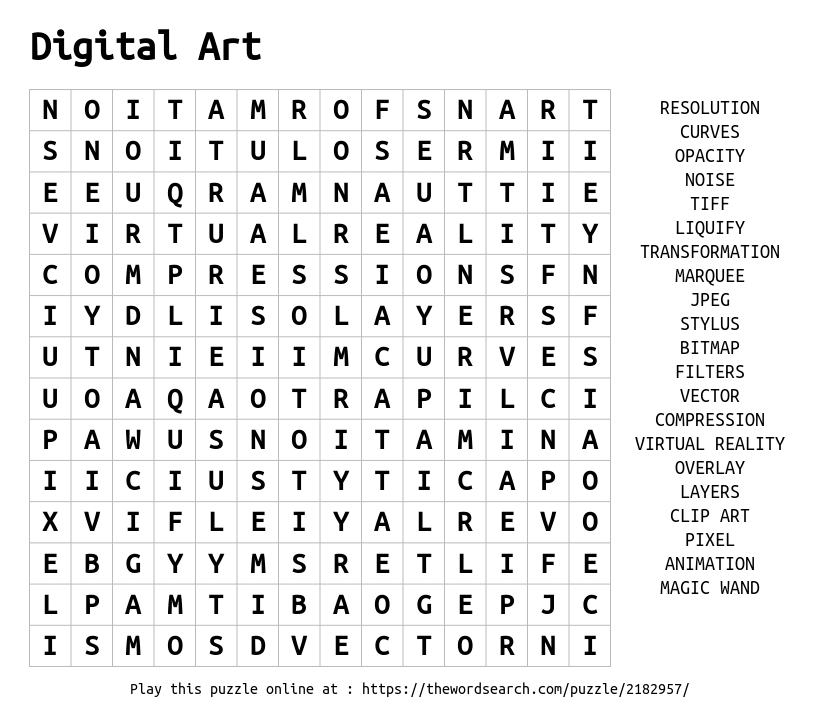The image depicts a black-and-white word search puzzle focused on digital art terminology. The entire background is white, and at the very top of the image, the text "DIGITAL ART" is prominently displayed in a basic font, resembling Times New Roman, in black lettering. Below this title is a grid resembling graph paper, consisting of approximately 15 rows across and 20 rows down, filled with black letters inside each box. To the right of this grid, there is a neatly centered column listing various digital art-related terms in capital letters, including: RESOLUTION, CURVES, OPACITY, NOISE, TIFF, LIQUIFY, TRANSFORMATION, MARQUEE, JPEG, STYLUS, BITMAP, FILTERS, VECTOR, COMPRESSION, VIRTUAL REALITY, OVERLAY, LAYERS, CLIPART, PIXEL, ANIMATION, and MAGIC WAND. At the bottom of the image, there's a smaller text that reads, "Play this puzzle online at https://thewordsearch.com/puzzle/2182957/".